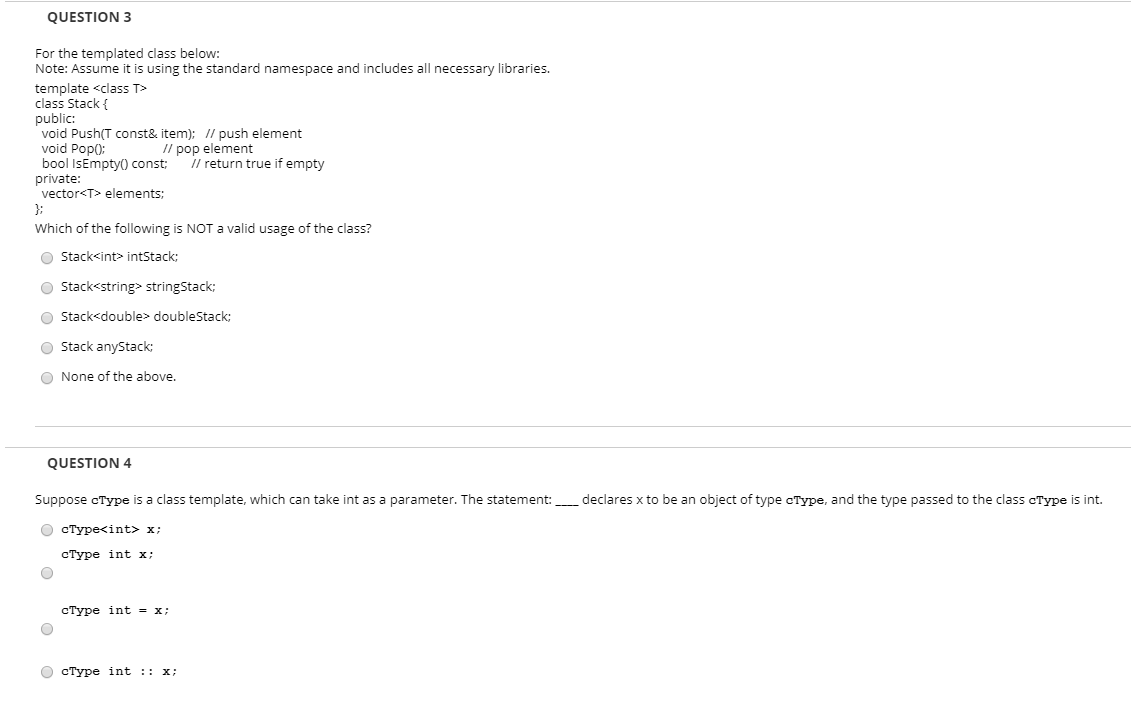In this image, the background is entirely white. At the top, there is black text in all capital letters reading "QUESTION 3." Below this, the text states, "For the templated class below, assume it is using the standard namespace and includes all necessary libraries." 

Under this instruction, a paragraph of black text describes a question, "Which of the following is not a valid usage of the class?" Following this, there are five different options labeled with circular selection markers, allowing a choice for the answer. The fifth option is "None of the above," also in black text. 

Beneath the options, two thin gray lines are visible, separating this question from the next. Below these lines, another prompt in all capital letters, "QUESTION 4," is written in black. The text under this heading reads, "Suppose a type is a class template which can take int as a parameter. The statement declares x to be an object of type and then the type passed to the class type is int." 

Below this explanation, there are four more options, each with a light gray circle next to it, indicating possible answer choices.